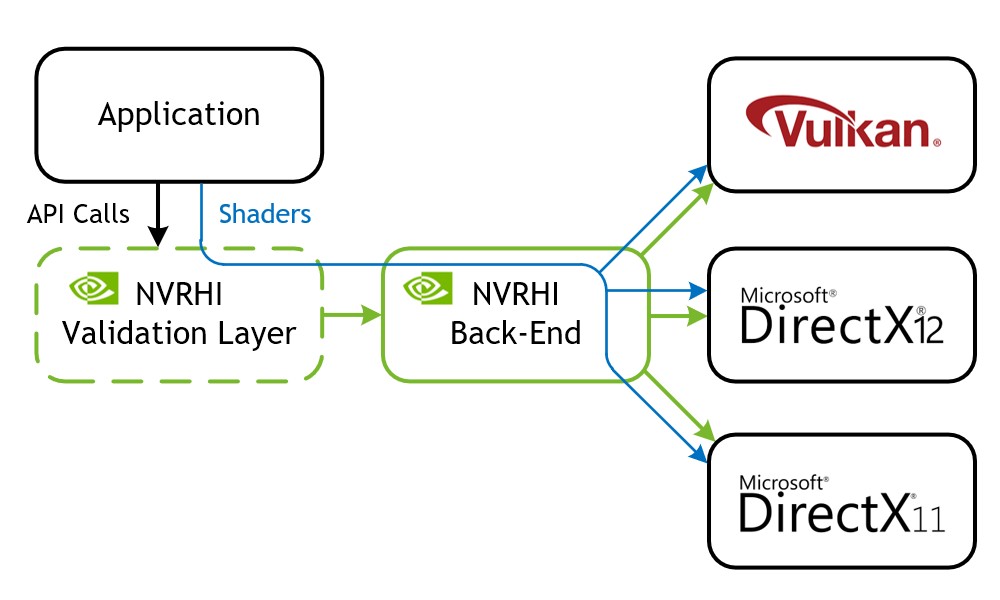The diagram is a detailed flowchart illustrating the pathway of graphical data through various layers and interfaces. On the far left, it begins with the 'Application' box, which sends 'API Calls' into the 'NVRHI Validation Layer,' outlined in a dotted green line and featuring a video symbol. The flowchart also depicts a blue line labeled 'Shaders' coming from the 'Application' box.

Next, the data moves from the 'NVRHI Validation Layer' to the 'NVRHI Backend'. The 'NVRHI Backend' then connects to three distinct pathways: 'Vulkan,' 'Microsoft DirectX 12,' and 'Microsoft DirectX 11.' Each of these layers, representing different graphical interfaces, takes input from the 'NVRHI Backend,' which is fed from the initial 'NVRHI Validation Layer'. The entire structure is organized into three horizontal layers from left to right, summarizing the flow from the application level through the backend, and finally into the various graphics APIs for rendering.